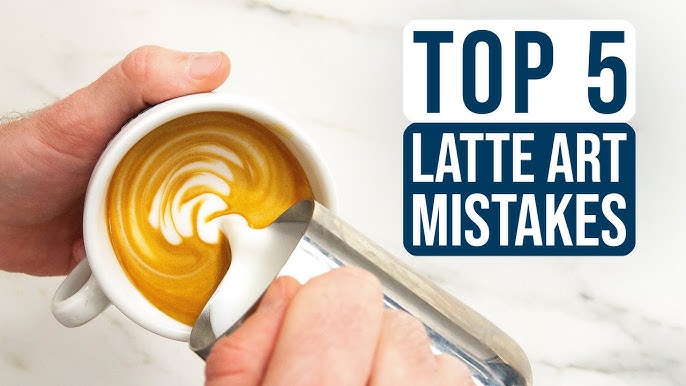In this detailed color image, a barista's hands are seen crafting a latte with a swirl design. One hand steadies a white cup filled with coffee, while the other hand pours cream from a silver pitcher, creating intricate latte art. The scene unfolds on a pristine white marble countertop, providing a clean and elegant backdrop. At the top left of the image, text boxes are visible: a white box with bold blue letters stating "Top 5," and directly below it, a dark blue box with bold white letters reading "Latte Art Mistakes." These indicate that the image is part of a guide or article focusing on common errors in latte art. The color scheme is predominantly white and blue, with hints of brown from the coffee, creating a visually appealing and informative snapshot.